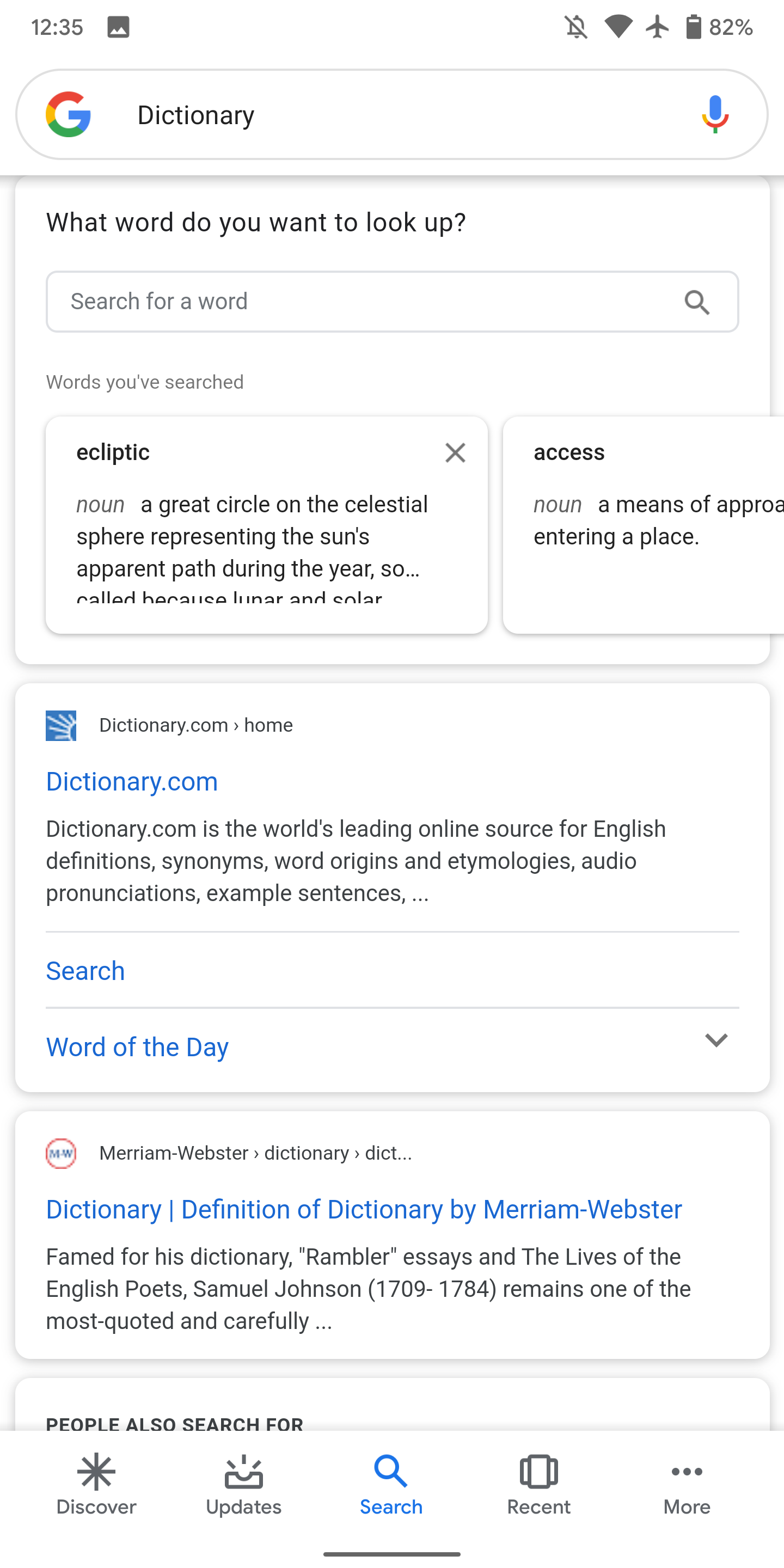This image captures a screenshot from a mobile phone displaying a Google search for the term "dictionary." At the top of the screen, Google prompts the user with the question, "What word do you want to look up?" Below this prompt is a text box where users can input their search terms. However, no word has currently been entered in the search box.

Beneath this, a section labeled "Words you've searched" displays previously searched terms. The word "ecliptic" appears first, defined as a noun: "a great circle on the celestial sphere representing the sun's apparent path during the year, so ...," with the remaining text cut off. Another previously searched term, "access," is listed next and defined as a noun: "a means of approach ...," with the definition also truncated.

Further down the page, links to additional dictionary resources are shown. One link directs users to Dictionary.com, offering options to search the site or explore the "Word of the Day." Another link leads to the Merriam-Webster dictionary entry for "dictionary," with the title "Dictionary Definition of Dictionary by Merriam-Webster."

This detailed snapshot highlights the user's interaction with Google and dictionary resources, showcasing their exploration of word definitions and search functionalities.